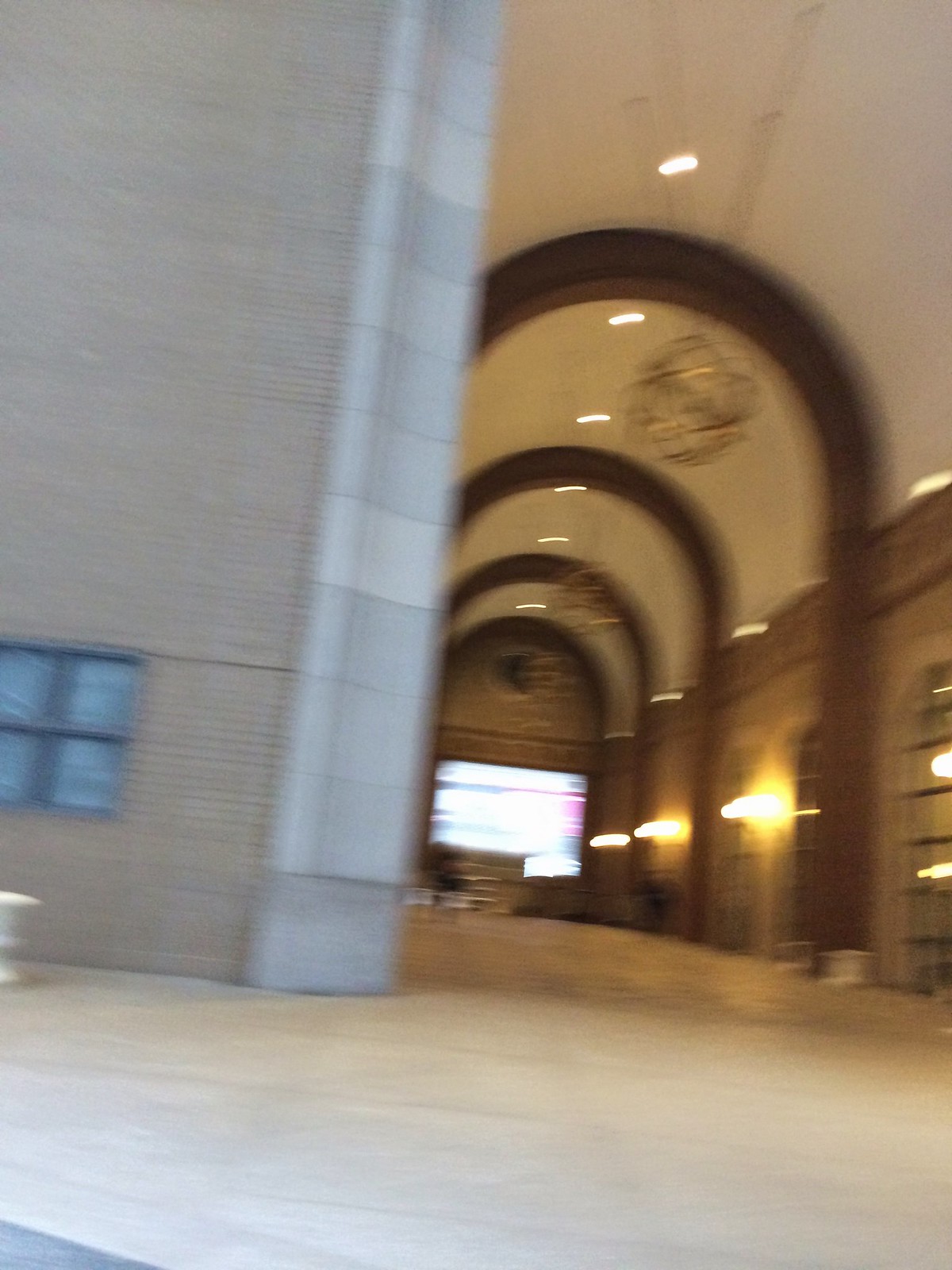The image captures a blurry and shaky photograph that appears to be taken while the person was running. The focal point is a hallway with a strikingly high ceiling. To the left, a tall brick wall adorned with a window featuring a black frame extends upwards. A significant feature is the gray stone molding that shapes the window. On the right, an expansive alleyway unfolds, accentuated by semi-circular wooden pallets and grand chandeliers. The high arches of the interior ceiling are white with dark brown supports, lit by both yellow and white lights. Further down the hallway, the cream or beige tiled floor, blended with hints of brown and other colors, leads to a brightly lit back area that remains indistinct due to the image's blurriness. The overall ambiance suggests a hotel reception area, enhanced by tan brick exterior elements and a mix of intricate brickwork. The ceiling also hosts a hollow, metallic, goldish globe, adding to the elegant decor.